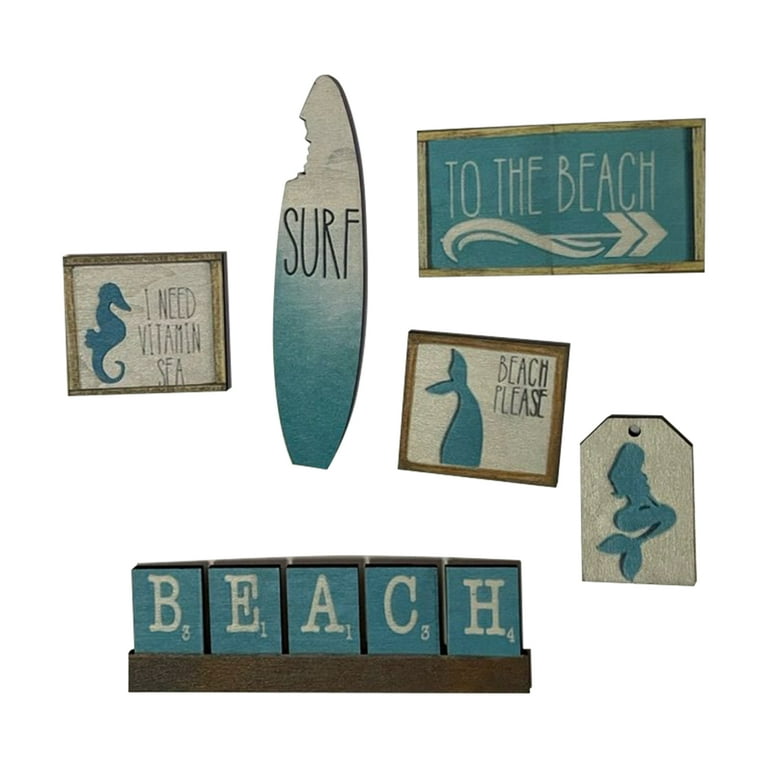The image showcases a collection of beach-themed decorations, perfect for home display. At the center, a framed picture with a blue silhouette of a seahorse playfully declares, "I need Vitamin SEA," with a pun on the word sea. Next, a surfboard in a gradient from white to blue appears bitten at the top, giving the impression of a shark attack, and it boldly states, "Surf." Another framed piece, featuring a teal background and white text, points "To the Beach" with a directional arrow, all enclosed in a yellow-brown wooden frame, similar to the seahorse picture.

Additionally, there's a frame with a white background showcasing a whimsical tail of either a fish or dolphin with the cheeky phrase, "Beach please." Close by, a photo with a white-grayish background highlights a beautiful teal silhouette of a mermaid. Further complementing the display is a Scrabble-style arrangement spelling out "Beach," with each letter on individual wooden tiles marked with their corresponding point values: B3, E1, A1, C3, H4, all on a white background, indicating professional production quality.

Lastly, there's an object resembling a luggage tag, featuring a blue mermaid, tying all the elements together with a consistent beach-inspired theme.